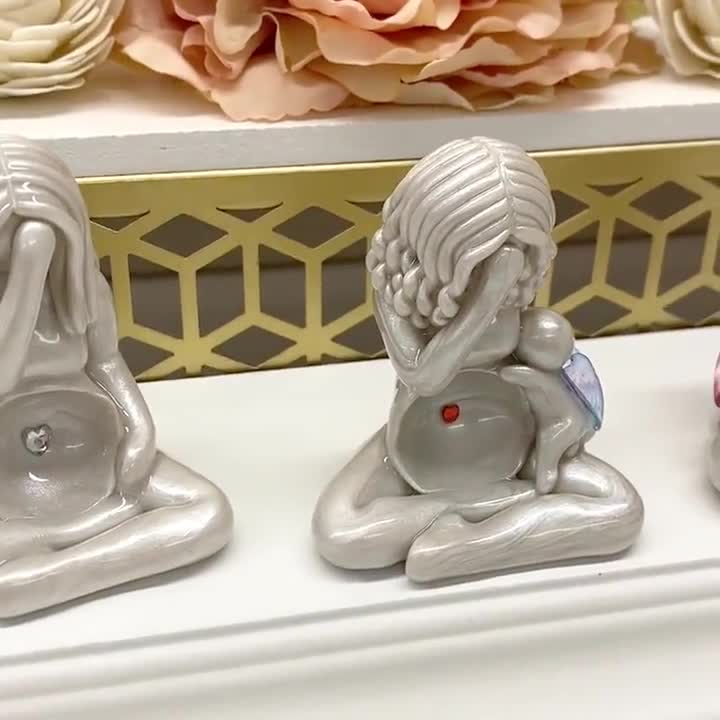This image showcases a pair of meticulously crafted sculptures displayed on a polished white wooden shelf. The primary sculpture, positioned near the center, depicts a woman seated cross-legged with a forlorn expression. Her detailed, wavy silver hair cascades forward as she bows her head, her right hand covering her face in apparent grief. Her left arm rests across her lap. At her midsection is a recessed circular medallion, featuring a vibrant red jewel, symbolizing a heart. Clinging to her neck and torso is a small infant with angel wings, indicating a poignant theme, possibly maternal sorrow.

To her left, an accompanying sculpture mirrors the primary figure's pose and distress. This woman, also seated cross-legged, has a less elaborate hairstyle and no infant at her side. The midsection of this figure also features a circular medallion, but with a silver heart instead. Both statues emit a high gloss finish, giving them a pearly, almost metallic appearance that contrasts with their somber mood.

Behind the figures is a backdrop of gold, comprised of a metal grate with a hexagonal pattern. Above this, partially visible, is another white wooden shelf adorned with delicate paper or origami flowers, adding a subtle element of nature to the composition. Overall, the image captures a solemn artistic presentation with intricate detailing and emotional depth.